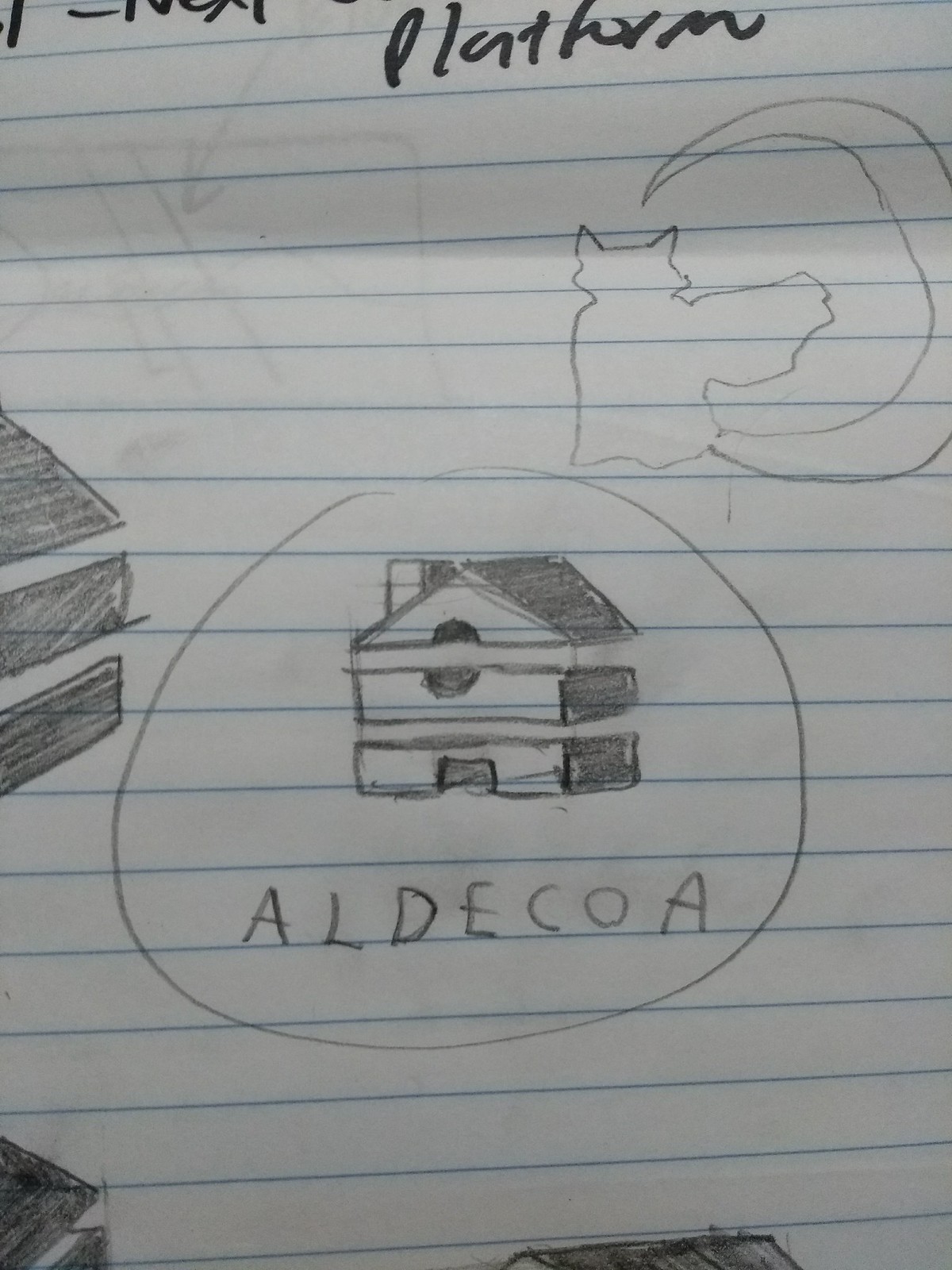The image features a detailed pencil drawing on a sheet of notebook paper, distinguished by its characteristic white background and blue horizontal lines typically seen in loose-leaf or notebook paper. Central to the drawing is a house, meticulously segmented into three distinct parts: the bottom, middle, and top sections. Below this segmented house is the word "A-L-D-E-C-O-A," written clearly in pencil. Encircling part of the house and the word beneath it is an incomplete pencil-drawn circle. To the top right of the house, there is an additional whimsical drawing, possibly of a kitten wearing a cape, accompanied by the outline of a crescent moon. While most elements in the drawing seem to extend beyond the visible area captured in the image, the focal points—the segmented house, the word "A-L-D-E-C-O-A," and the kitten with the crescent moon—remain prominently displayed at the heart of the composition.